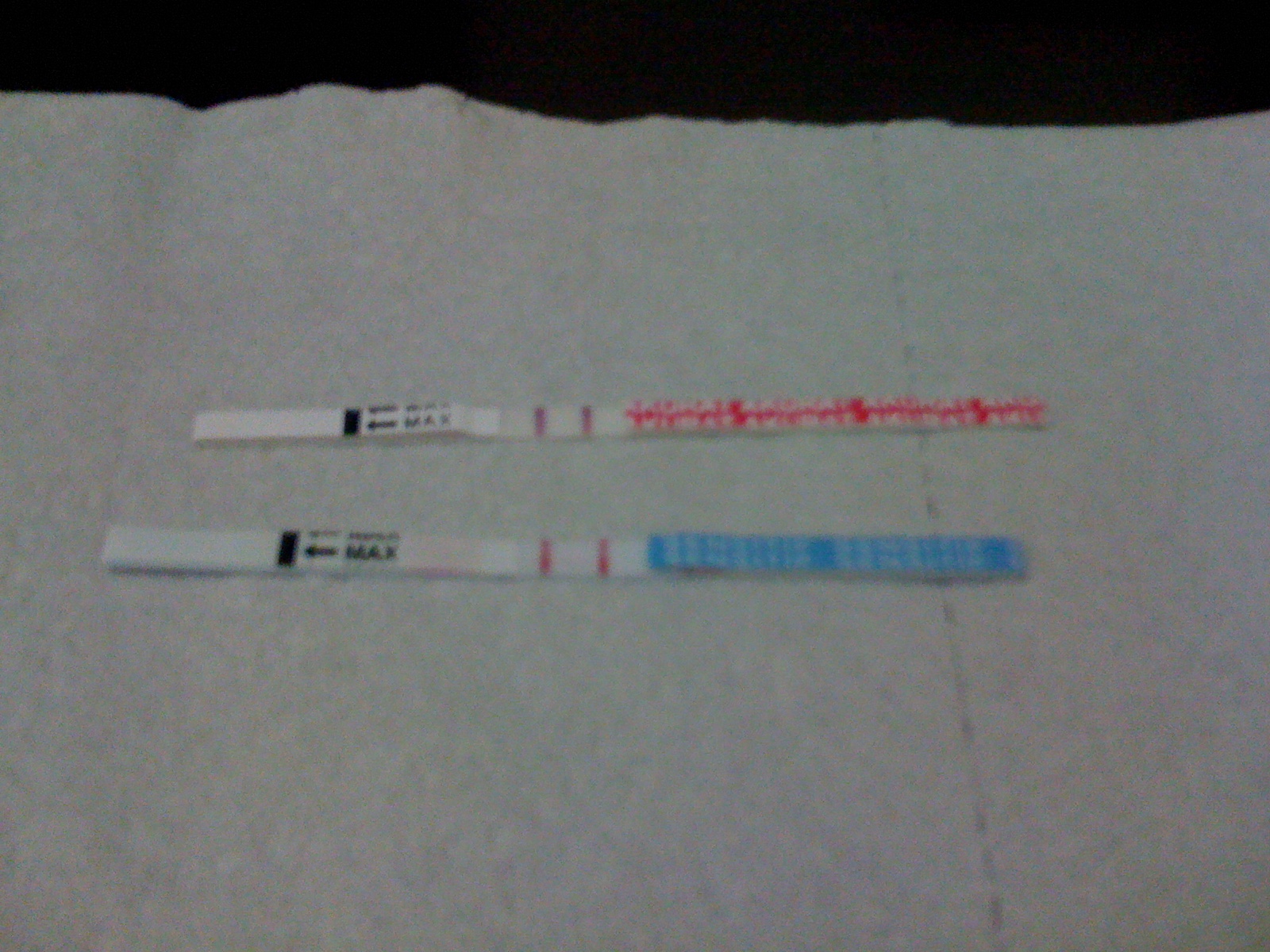This is a color photograph taken in dim lighting, making the image slightly out of focus. The majority of the photo is occupied by a white surface that appears more grayish with subtle variations in color, including hints of purplish and greenish tones. This surface, possibly cloth or paper, has a somewhat textured appearance. The background of the image, located at the very top, is entirely black, suggesting that the white surface might be placed on a dark table.

Prominently displayed on this surface are two very thin, long strips that seem to be made out of plastic. The strip positioned towards the top of the image is predominantly white with pink designs. It features some bold black writing on the left side, although it is too out of focus to be readable. The adjacent strip is similar in shape and size but differs in color, showcasing a turquoise blue and white pattern instead of pink and white.